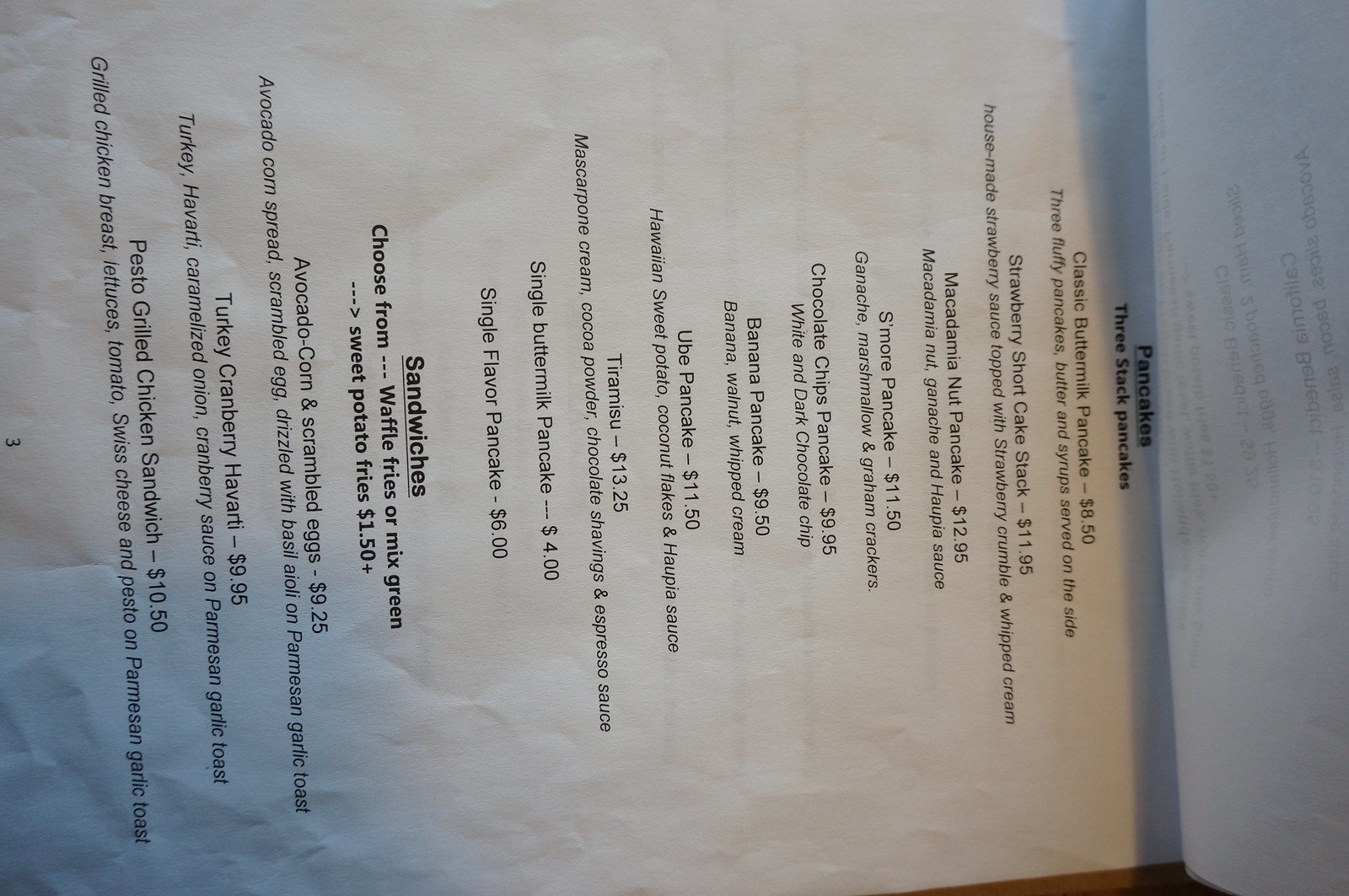A photograph depicts a white piece of paper, oriented sideways with the top of the page on the right side of the image and the bottom on the left. This piece of paper is crinkled, indicating frequent use, and appears to be the second page of a restaurant menu secured on a clipboard, with the first page slightly lifted and barely visible on the right edge of the frame.

The menu page prominently lists an array of pancake options at the top, beginning with "Three Stack Pancakes," followed by various meticulously described pancake varieties and their corresponding prices, ranging from approximately $8.50 to nearly $14. The offerings include:

- Classic Buttermilk Pancakes
- Strawberry Shortcake Stack
- Macadamia Nut Pancake
- S'more Pancake
- Chocolate Chips Pancake
- Banana Pancake
- Ube Pancake
- Tiramisu Pancake
- Single Buttermilk Pancake
- Single Flavor Pancake

Beneath the pancake selection, there is a smaller section dedicated to sandwiches. This section provides a choice between waffle fries or mixed greens, with the option to substitute sweet potato fries for an additional $1.50. The sandwich offerings, priced around $9 to $10 each, include:

- Avocado Corn and Scrambled Eggs
- Turkey Cranberry Havarti
- Pesto Grilled Chicken Sandwich

The neatly organized and detailed descriptions offer a glimpse into the restaurant's diverse and appetizing menu options.